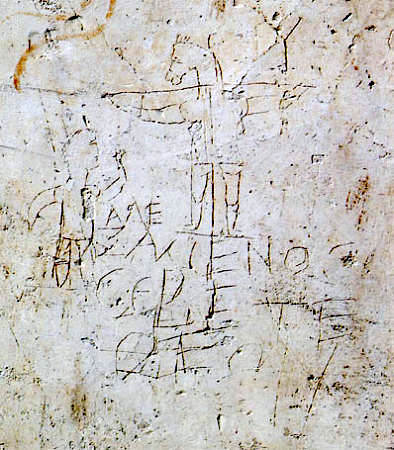In this image, the focus is a weathered, light brown wall marred with patches of brown dirt and grime. The surface of the wall is intricately carved with various figures and markings. Dominating the center of the wall is an elaborate carving of a mythical figure: a creature with the body and limbs of a human, but the head of a horse and large, widely spread wings extending from its back. This horse-headed figure, with its gaze directed towards the left side of the image, exudes an aura of ancient mystique.

To the lower right of the horse-headed figure, the letters "N-O" are conspicuously etched into the wall. To the left of the central figure stands a smaller carving of a person approaching the horse-headed being, carrying an indistinct object, which seems to be the reason for the horse-headed figure's keen attention. The wall is further adorned with several other carvings, though their details are indistinct and less discernible. This scene captures a moment that seems frozen in time, enveloped in mystery and ancient artistry.